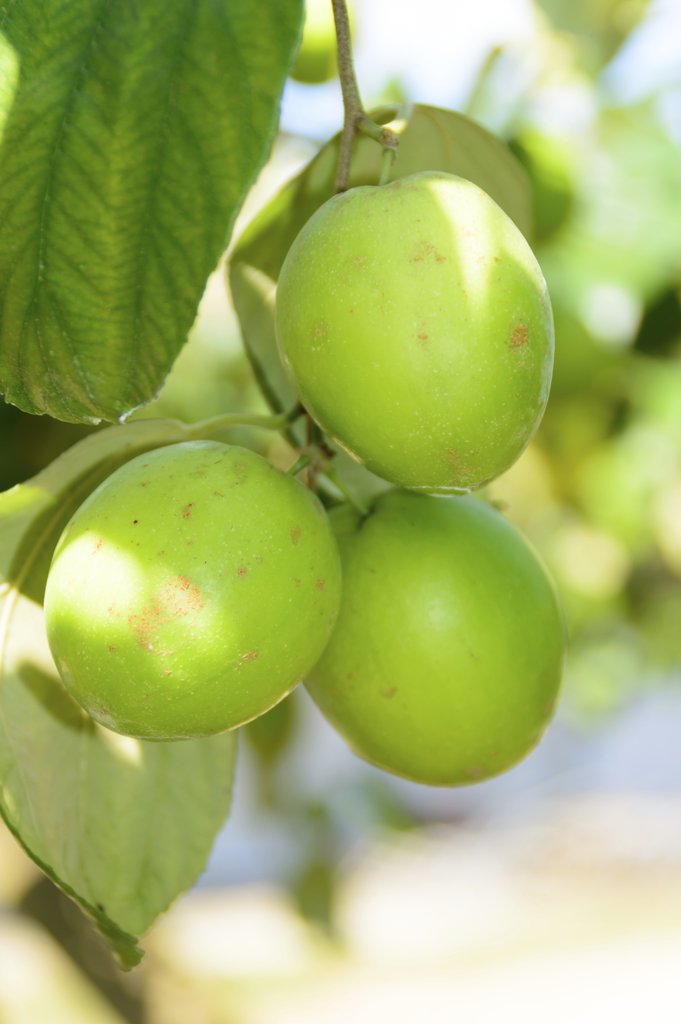The image depicts a close-up of three green, oval-shaped fruits or beans hanging on a tree, possibly resembling limes, against a backdrop of highly blurred foliage with light dappling through. Taken during the daytime, the fruits exhibit small brown spots and a shaft of sunlight glistens on the top fruit. The fruits are surrounded by large green leaves, some of which are as large as the fruits themselves, with additional leaves filling the background. Spaces between the leaves reveal glimpses of blue sky, enhancing the outdoor setting. The textural details of the fruits and leaves are sharp, contrasting with the cream-colored and blurred background which suggests a bright, sunny day.